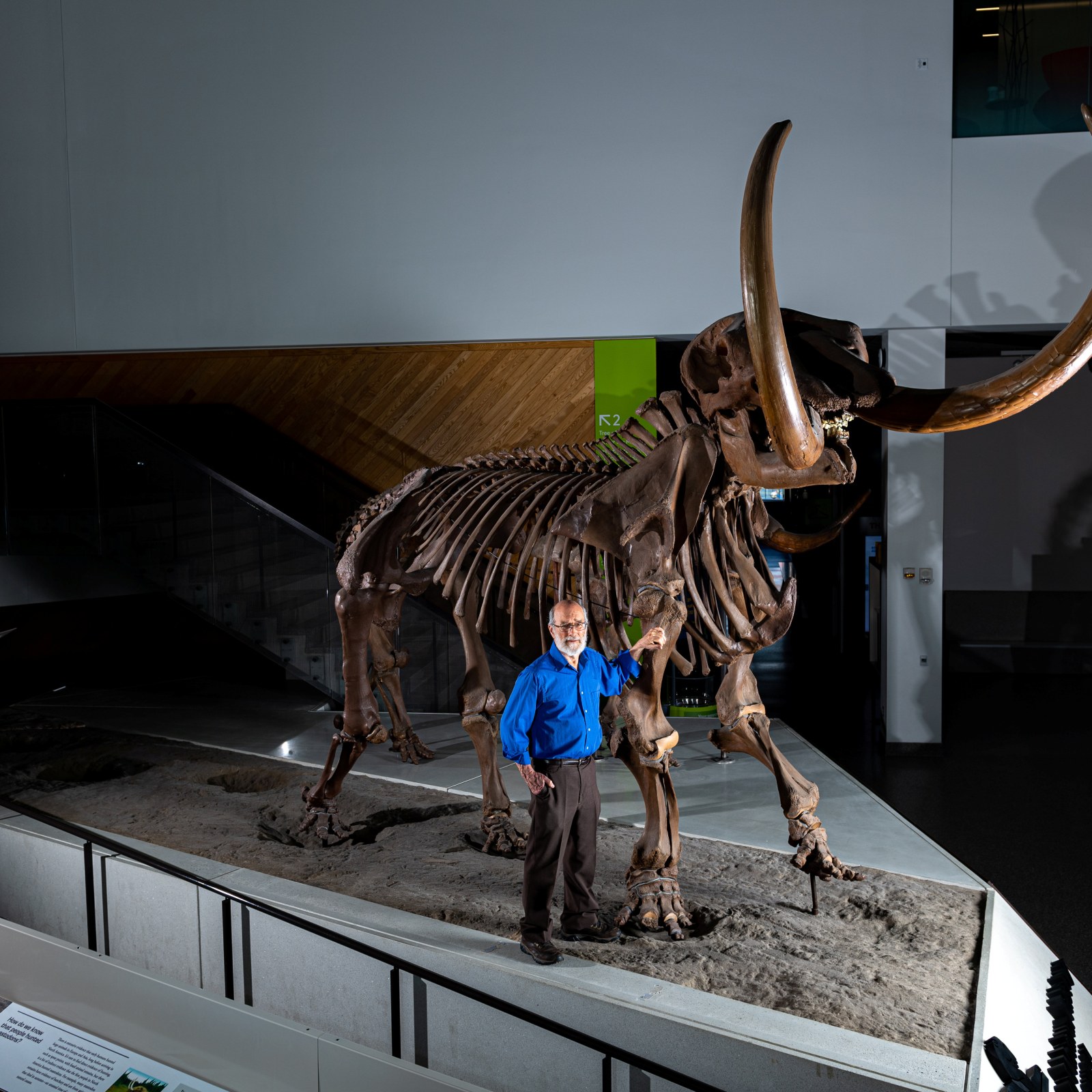This photograph, taken inside a science museum, prominently features the intricate skeleton of a mammoth displayed on a mound of dirt, surrounded by a marble barrier to prevent visitors from touching it. The impressive fossil, with its detailed spine, ribcage, legs, and large, protruding tusks, stands majestically as the focal point of the image. In the background, we see a white wall transitioning into a wooden section with stairs leading to the second floor, indicated by a green line with an upward arrow and the number '2'. An older, bald man with a white beard and glasses, dressed in a blue button-up shirt and dark pants, stands beside the mammoth. He has one hand in his pocket while the other rests on the mammoth's front leg. His presence, only reaching up to the mammoth's chest, highlights the enormous size of the mammoth. The gentleman appears to be posing for the camera, adding a human element to this grand prehistoric display.